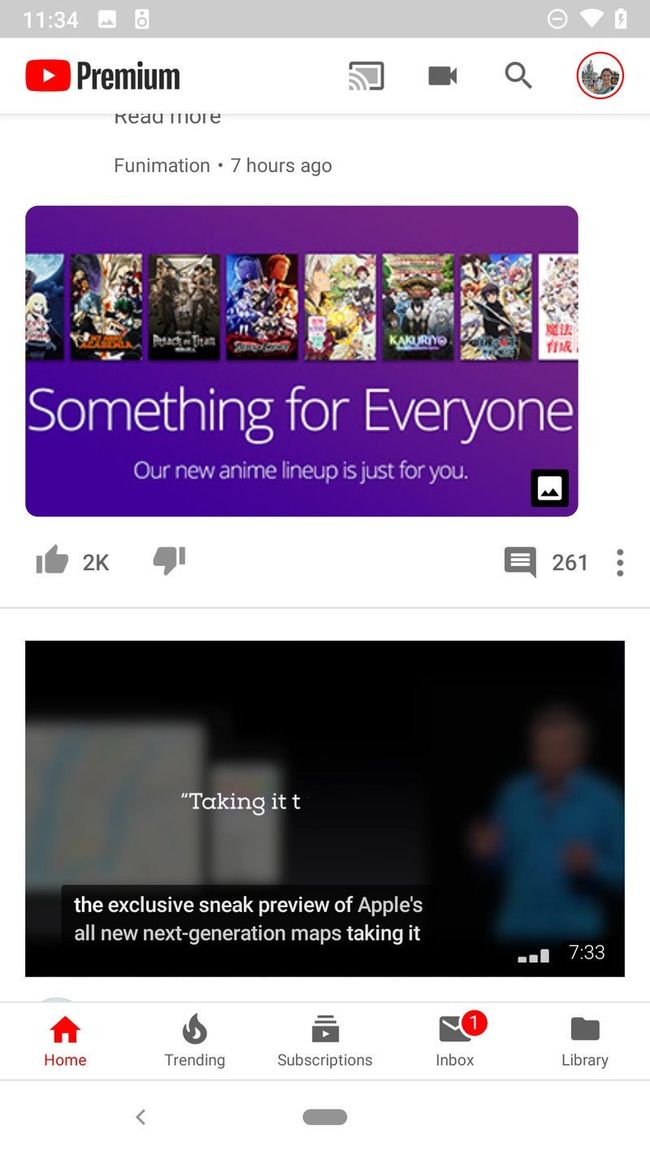An image depicts a smartphone screen displaying the YouTube Premium interface. At the top, the "Premium" label is prominently featured next to the YouTube logo, set against an otherwise predominantly white background with red accents typical of YouTube's design. On the screen, there are two main images from video thumbnails.

The first thumbnail has a duration of 7 minutes and 33 seconds and is titled "Exclusive Sneak Preview of Apple's Next Generation Maps," related to an Apple event or update. The second thumbnail belongs to the channel 'Funimation,' showcasing a promotional screen capture that reads, "Something for everyone, our new anime lineup is just for you," accompanied by an array of anime cover art.

At the bottom of the interface, the navigation bar displays icons for Home, Trending, Subscriptions, Inbox, and Library. There is a notification indicating one unread message in the Inbox. The user's profile picture shows a young individual whose exact gender is indiscernible; they appear to be in a European outdoor setting, possibly near an old building. Additional interface elements include a Chromecast button, a video camera button, and a search button.